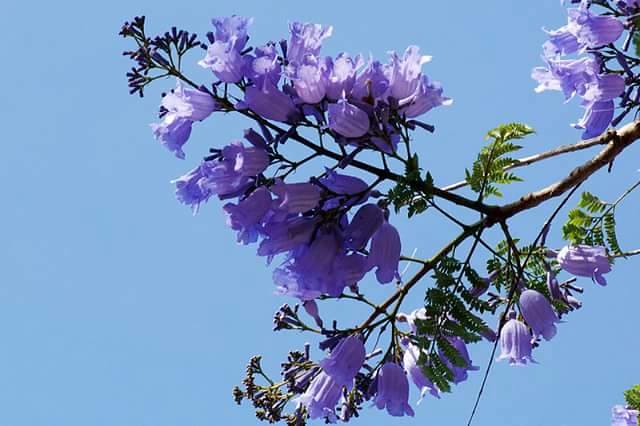This captivating photo captures the delicate beauty of a tree branch adorned with clusters of lilac purple flowers set against a pristine, cloudless blue sky. The perspective of the shot seems to be from below, looking up, highlighting the contrast between the vivid colors of nature and the clear backdrop. The flowers, appearing lightweight and ethereal, dangle gracefully from the tips of the branches, suggesting they are in the midst of blooming, likely indicating an early spring setting. The green leaves are scattered throughout the branches, providing a lush frame for the profusion of blossoms. The main tree limb, portrayed with its dark wooden texture, extends diagonally with multiple smaller offshoots, each festooned with these vibrant flowers and budding tips. Though the exact species of the plant remains unidentified, the scene exudes a serene and tranquil ambiance, capturing a perfect moment of natural beauty in full bloom.